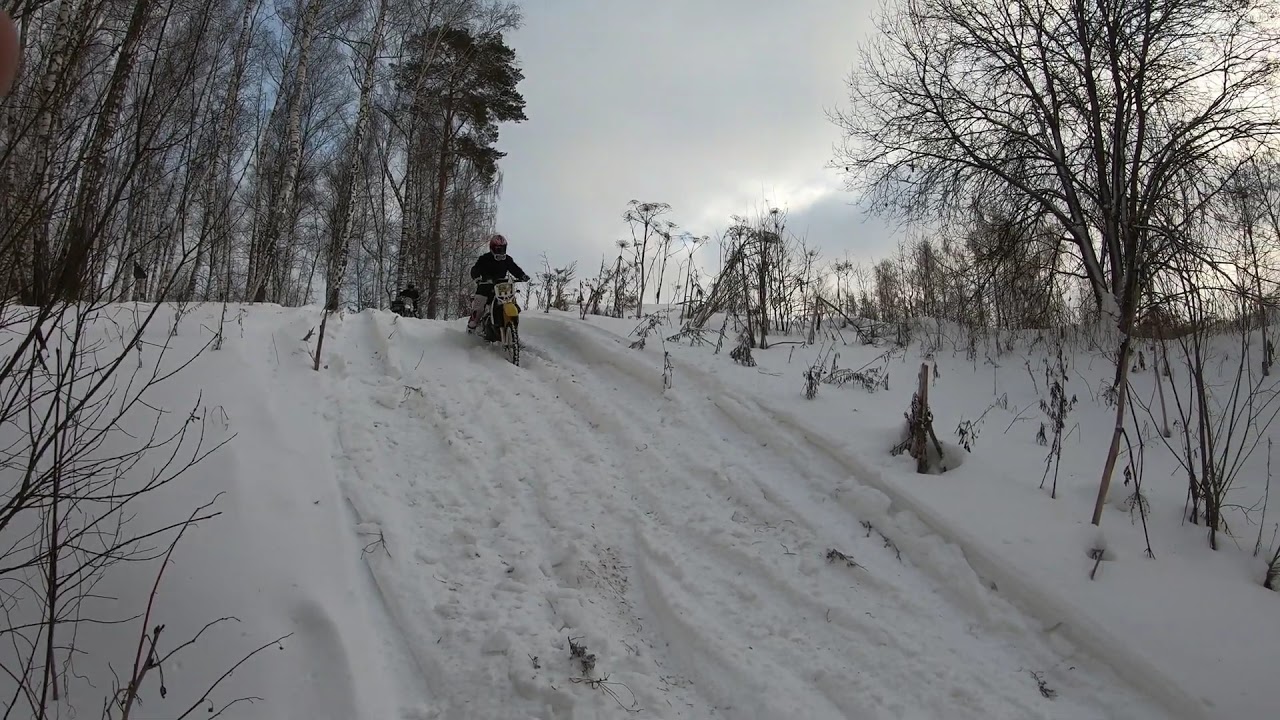This image showcases a snowy outdoor scene dominated by barren trees and an overcast, dark gray sky. The focal point is a dirt road with a dirt biker descending a small hill. The biker in the foreground is riding a yellow and black motorcycle and is dressed in a black jacket with a yellow helmet. Snow blankets the ground, broken up by the dirt road winding through the landscape. A second biker is visible in the distance, riding a black motorcycle and wearing a black jacket with a black helmet. The surroundings are filled with various trees and shrubs, mostly devoid of leaves, adding to the stark, wintry atmosphere.